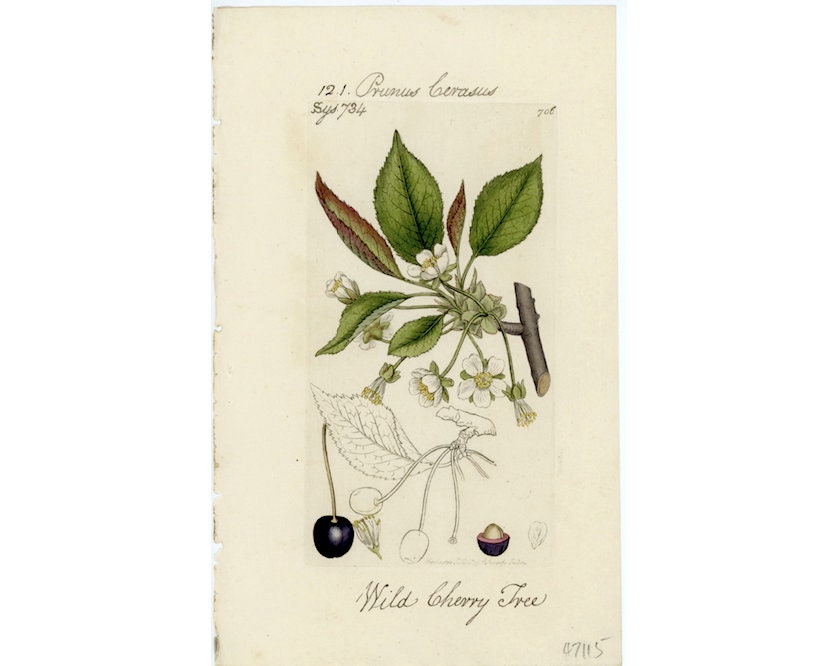This illustration, reminiscent of an antique botanical print, depicts a "wild cherry tree" and features detailed artwork on an off-white, slightly aged page. Centered on the page is a vibrant drawing of a branch with several green leaves and white, five-petaled flowers with yellowish cores. Some of the leaves exhibit a reddish-brown hue. Just beneath this primary image is a black and white pencil sketch that appears to show a different developmental stage of the plant, with distinct bulbous formations instead of flowers, and a black cherry prominently rendered in color beside it. Adjacent to this sketch is a smaller, detailed image that might depict a half-cut almond. The topmost part of the page, labeled "12.1", includes cursive writing that is difficult to decipher, but seems to say "prunus carasus". Below, additional text reads "SYD 734" along with other less clear numerals and characters. At the very bottom right, a handwritten annotation in pencil marks "47115". This detailed arrangement of botanical elements captures the timeless essence and intricate study of the wild cherry tree species.